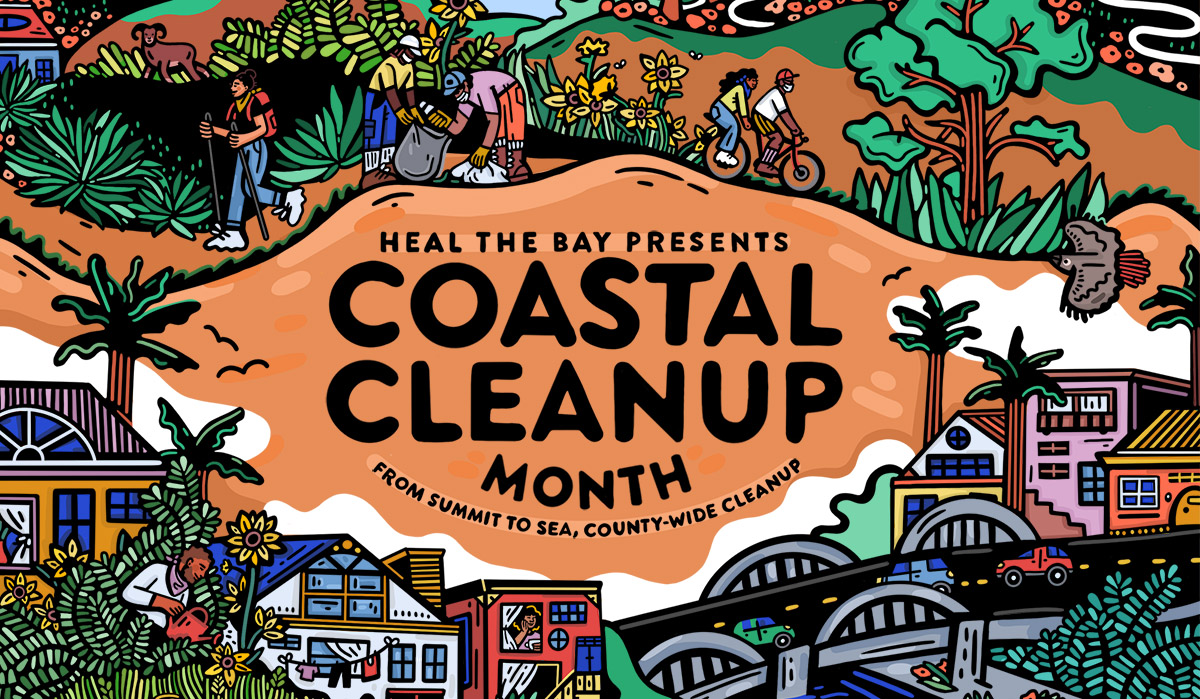This detailed outdoors drawing, designed as a graphic for an advertisement, showcases a vibrant scene for an event. In the center, a text overlay reads, "Heal the Bay presents Coastal Cleanup Month, from Summit to Sea, Countywide Cleanup." Adjacent to the word "Coastal" is an illustration of a bird. The imagery is divided into two primary sections: a mountainous and woodland area above, and a bustling town scene below.

At the top, a prominent mountain serves as the focal point. People are seen biking down its slopes while, at a lower elevation, two individuals in colorful attire—yellow and pink—are actively picking up trash with gray bags. To the left, a hiker in blue jeans and a red backpack is trekking with walking sticks through a lush forest adorned with green grass, trees with brown trunks, and vibrant flowers in shades of yellow and pink. 

Below this natural landscape, the scene transitions into a lively town. To the left, a white building with a gabled roof stands next to another with a similar roof design. Between these buildings and stretching across a blue waterway is a bridge with arches, traversed by red, blue, and green vehicles. The town is dotted with palm trees, sunflowers, and a mix of colorful buildings, including a pink flat-roofed structure, an orange building, and another with a gabled roof. The inclusion of black and yellow road markings adds to the urban detail, while more palm trees with black and green hues frame the lower foreground.

This rich tapestry of natural beauty and urban life encapsulates the event's theme, advocating for community involvement in environmental cleanup from mountainous regions to coastal areas.